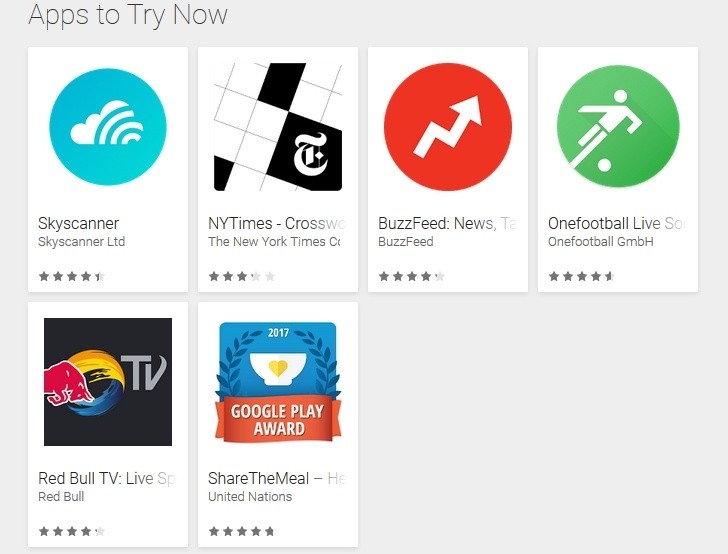The image features a light gray background with the heading "Apps to Try Now" in bold black print at the top. Below the heading, six app icons are displayed in a grid.

**Top Row:**
1. **Skyscanner**: Represented by a large blue circle with a cloud icon, labeled "Skyscanner LTD", boasting approximately four and a half stars.
2. **New York Times Crossword**: Feature a white background, rated at three stars.
3. **BuzzFeed News**: Displayed within a red circle with a jagged arrow, rated at four stars.
4. **One Football Live**: A green circle showing someone playing soccer or football, rated four and a half stars.

**Bottom Row:**
1. **Red Bull TV Live**: Shown within a black square featuring a red dog and additional orange and black elements, with "TV" printed in gray, rated at four stars.
2. **ShareTheMeal by the United Nations**: Displayed within a white background with blue and red colors and a "Google Play Award" emblem, nearly five stars.

The diverse collection of apps indicates a variety of utilities and interests, from travel and news to sports and philanthropy.